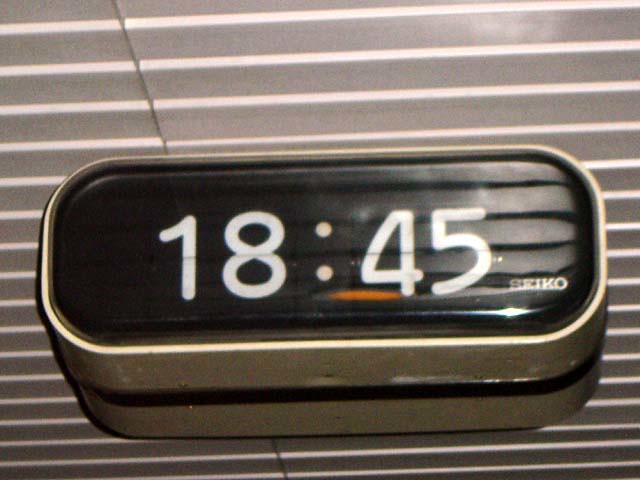This color landscape photograph features a small, unique flip clock made by Seiko, positioned on a tabletop that resembles a vent. The clock's design includes a metal, silver-colored rectangular frame with rounded corners. The clock face is black, displaying white numbers that read "1845." In the lower right corner, the brand "Seiko" is clearly visible. Adding a touch of character, there is a minor imperfection—a streak of orange below the number four, likely from paint wear. The background highlights white window shades that subtly accentuate the clock's presence.